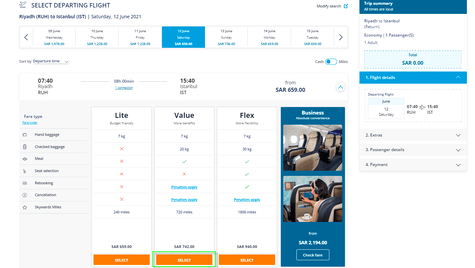The image depicts a section of a website dedicated to booking airfare, featuring a detailed layout for flight selection. Prominently displayed on the upper left, against a white background, is the header in bold, black text that reads "Select Departure Flight." To the upper right, there's an option labeled "Modify Search." Below this, in blue on white text, is a section titled "Trip Summary."

Underneath the headers, on the left-hand side, the flight route and date are specified, though the date is not completely legible. Below this, there are seven clickable options for selecting different dates. Each option is displayed in white text on a black background, with the exception of the fourth (center) option, which is highlighted in blue on white, indicating the selected date.

Further down, departure details are stated with "Departure 07:40AM" and "Arrival 15:40PM." The price is listed as "from SAR 650." 

On the left-hand side, continuing downwards, there is gray text on a black background, categorizing different fare plans. These include three plans: Light, Value, and Flex, each displayed in white on black text. At the bottom, yellow on orange buttons allow for class selection, with the chosen option being "Business Class" listed at a price of SAR 2,000 and change.